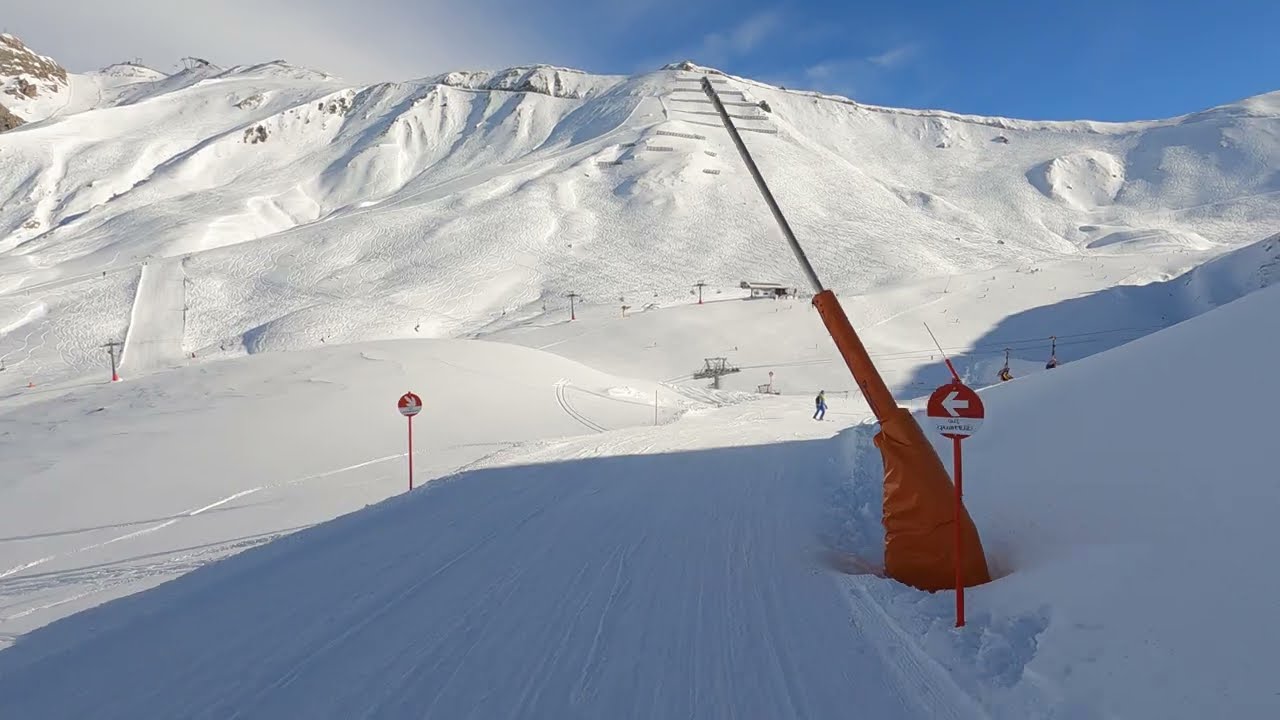This image captures a panoramic view of a pristine, snowy landscape, likely a ski resort, surrounded by snow-covered hills and mountain peaks. The sky above is a mix of bright blue and scattered white clouds, indicating a clear, sunny day.

In the foreground, the scene reveals a well-worn ski run. A flat, snowy area suggests a popular spot for skiing, with visible paths created by skiers. A red pole with a circular sign is positioned on the left side, though its details are unclear. On the right side, there's a vivid red base with a silver pole angled upwards, possibly indicating a gate or directional marker. Nearby, another sign with an arrow pointing left guides skiers, complementing the visible structure of a ski lift in the middle distance, with carts gliding across wires from left to right.

Further in the distance, scattered poles, possibly power lines or markers, punctuate the snowy expanse. A solitary figure, perhaps a skier or walker, is spotted on the path, heading deeper into the landscape. The untouched, smooth snow on the lower right slopes gently upwards, adding to the serene yet dynamic environment of this snow-covered haven.